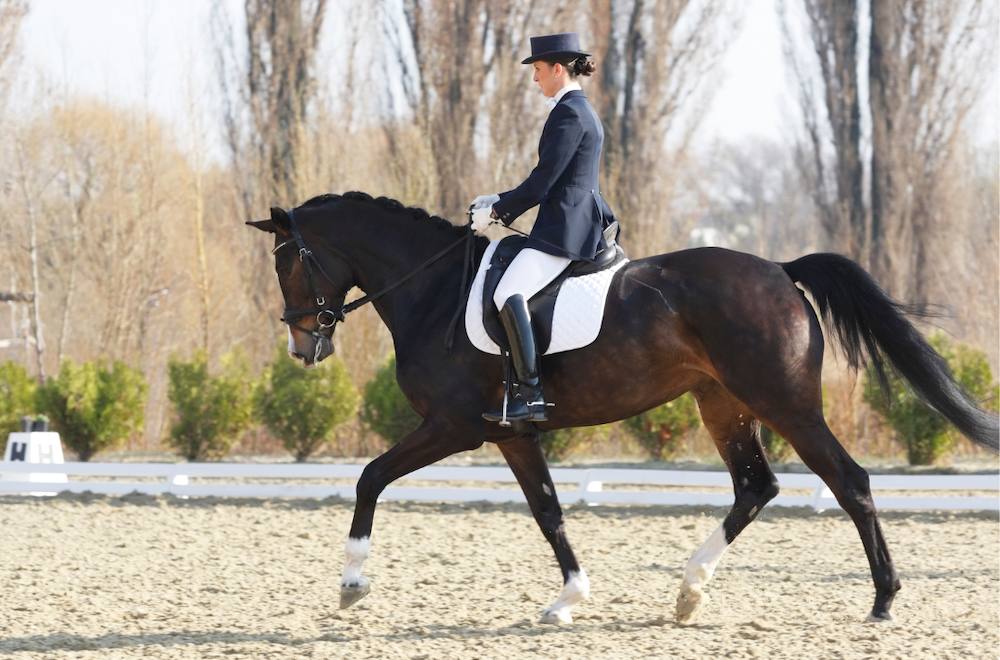In an outdoor scene with a yellow-colored sandy ground, a light-skinned woman sits astride a large dark brown horse that has a beautifully coiled black mane and a black tail. The horse is moving to the left with a slight prancing gait, its head down slightly, showcasing three white boot-like markings on its legs, leaving the left rear leg entirely brown. The horse wears a black saddle with a white saddle blanket beneath it. The rider, impeccably dressed in formal equestrian attire, wears a short-topped, broad-rimmed hat, a tailored dark blue jacket, white riding pants, tall black leather boots complete with silver-colored stirrups and spurs, and is further accessorized with white gloves. Her hair is neatly pulled back into a bun. She sits upright, holding the reins with her arms outstretched in front of her. A narrow, white fence runs near the ground in the background, bordered by a line of green short bushes and tall, sparsely-leaved trees.